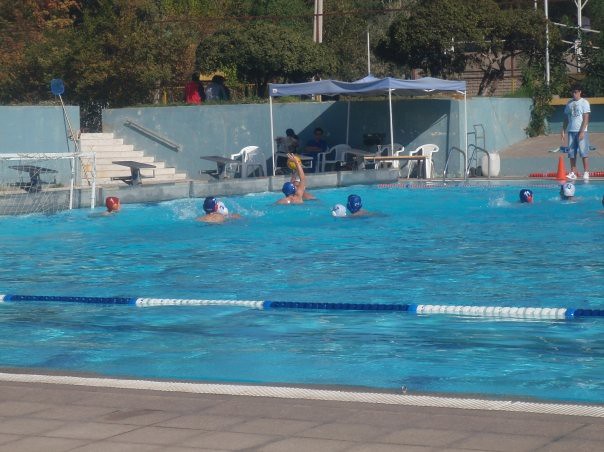The full-color photograph depicts a lively outdoor scene at a community swimming pool on a bright sunny day. The pool is surrounded by a walkway made of brown tiles, and the water shimmers a vibrant blue. There is a single plastic lane divider in the pool, likely for lap swimming. Dominating the scene is a water polo game, with several players actively engaged, wearing their respective caps—blue, white, and a goalie distinctively in red. Two players are prominently fighting for the ball in the center. On the far side of the pool, a gentleman dressed in a white shirt, blue jean shorts, and white shoes stands, possibly as a referee or lifeguard. In the background, shaded under a small canvas tent, a few spectators sit on white plastic chairs, intently watching the action. The scene is set against a backdrop of lush trees, enhancing the summery atmosphere of this vibrant, high-energy moment.